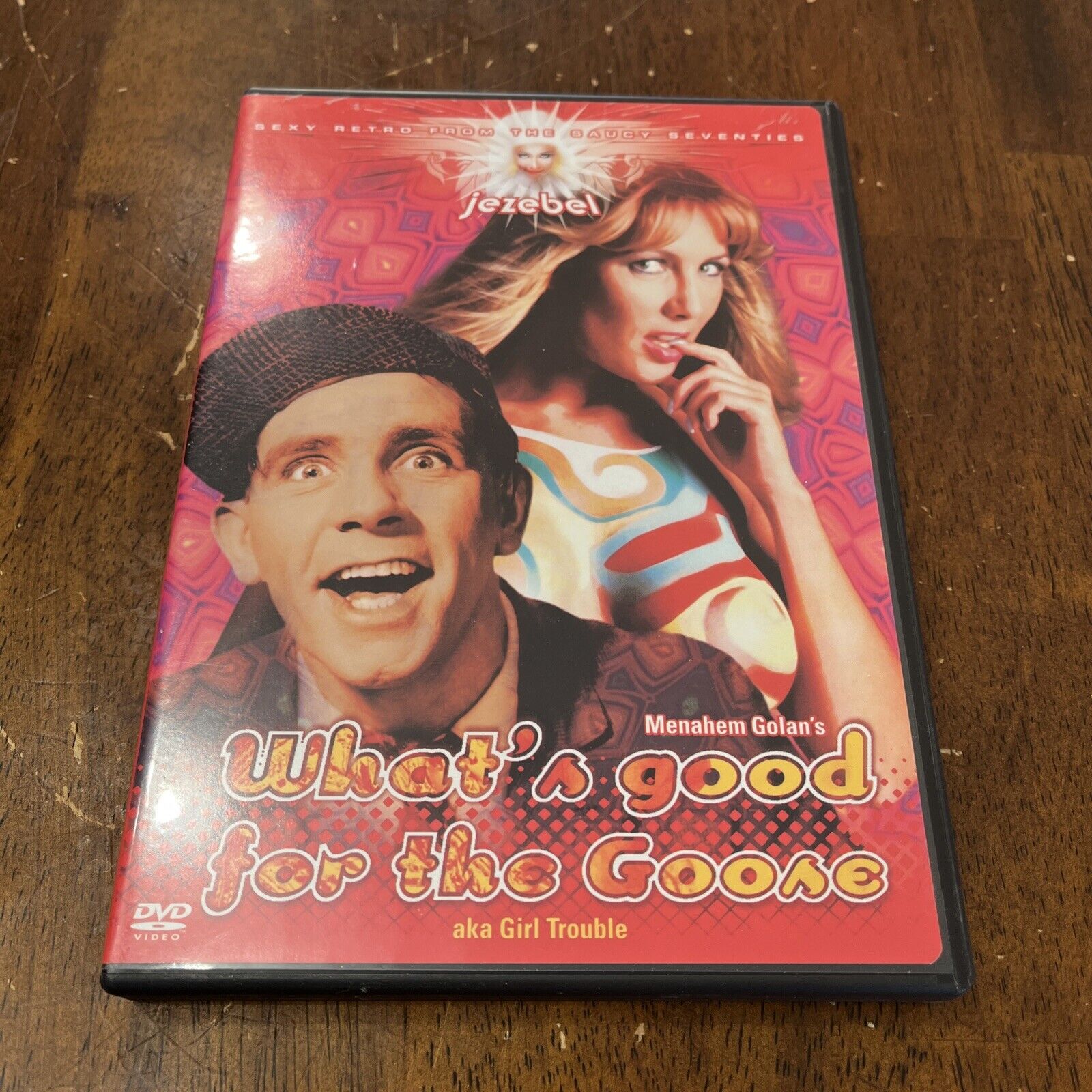The image showcases a detailed DVD cover set against a brown wooden surface. The cover prominently features the title "Jezebel" at the top, followed by the subtitle "Sexy Retro from the Saucy 70s" in smaller text. The names "Menahem Golan's What's Good for the Goose aka Girl Trouble" are also displayed towards the bottom. The overall design exhibits a 70s-inspired psychedelic theme with vibrant hues of pink, purple, orange, and green, and includes trippy squared and diamond patterns.

Front and center, the cover portrays two main figures: a man and a woman. The man, located off to the right, has a discolored, yellowish tint to his skin, wears a hat, and is dressed in a brown suit with a white-collared shirt. His mouth is open wide in an excited expression. The woman, prominently featured in front, is a Caucasian with long, wavy blonde hair, sporting red lips and some makeup. She bites her finger suggestively while looking forward. Her chest is painted with multicolored stripes—red, orange, blue, green, and white—with a distinctive circular red stripe around her breast. In contrast, the background behind these figures is a dynamic mix of retro and psychedelic elements, reinforcing the theme of the 1970s.